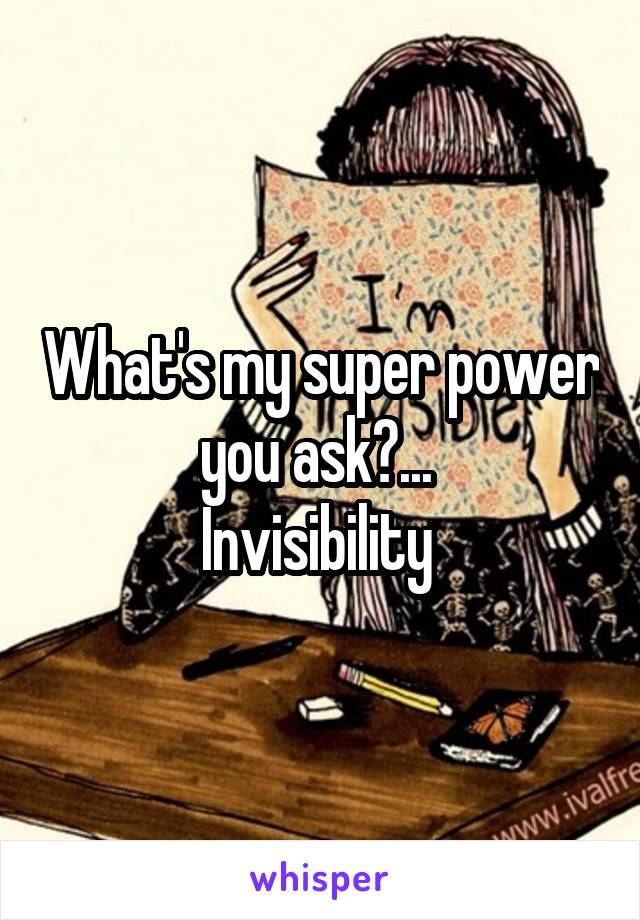In this detailed sketch drawing, a girl with pink, white, and black hair is sitting at a wooden, brown table. Her face is hidden behind a piece of paper adorned with pink and red roses and blue leaves on a white background, on which "I'm invisible" is written in black. She is dressed in a black shirt covered in white skeleton patterns. The table in front of her holds a pen, a pencil with a red eraser, a white rubber eraser, and a small notebook featuring an orange and black monarch butterfly. Partially visible on the side of the table is the URL www.ivalfre. Over the sketch, white text with a black outline reads, "what's my superpower, you ask... invisibility." Below the drawing, in the center, the word "whisper" is written in purple font.